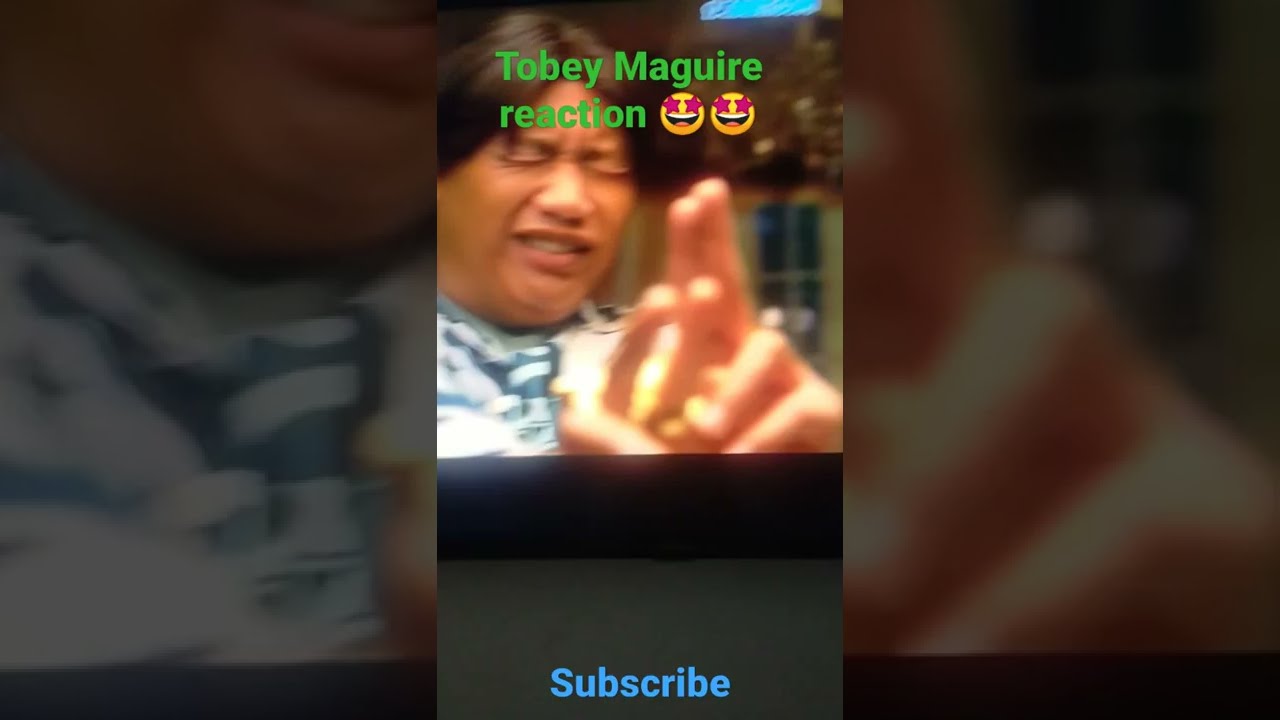The image consists of three parts with the central focus being a picture captioned "Tobey Maguire Reaction" in green text at the top. This shows an Asian male, with brown hair parted in the middle, scrunched eyes, and his mouth in a grimace, revealing his upper teeth. The man is wearing a blue shirt and appears to be posing in front of a house with a window behind him. His hands are raised, with the index and middle fingers on both hands pointed upwards, as if making a gesture towards the viewer.

On either side of the central image, there are vertical bands displaying zoomed-in segments of the same photograph. The left band shows a close-up of the man's face and the collar of his shirt, while the right band zooms in on his hands and part of the background, which includes a window and a deep brown trim. Purple-star-eyed smiley emojis accompany the green text at the top, and a blue "subscribe" text is prominently featured at the bottom against a gray background.